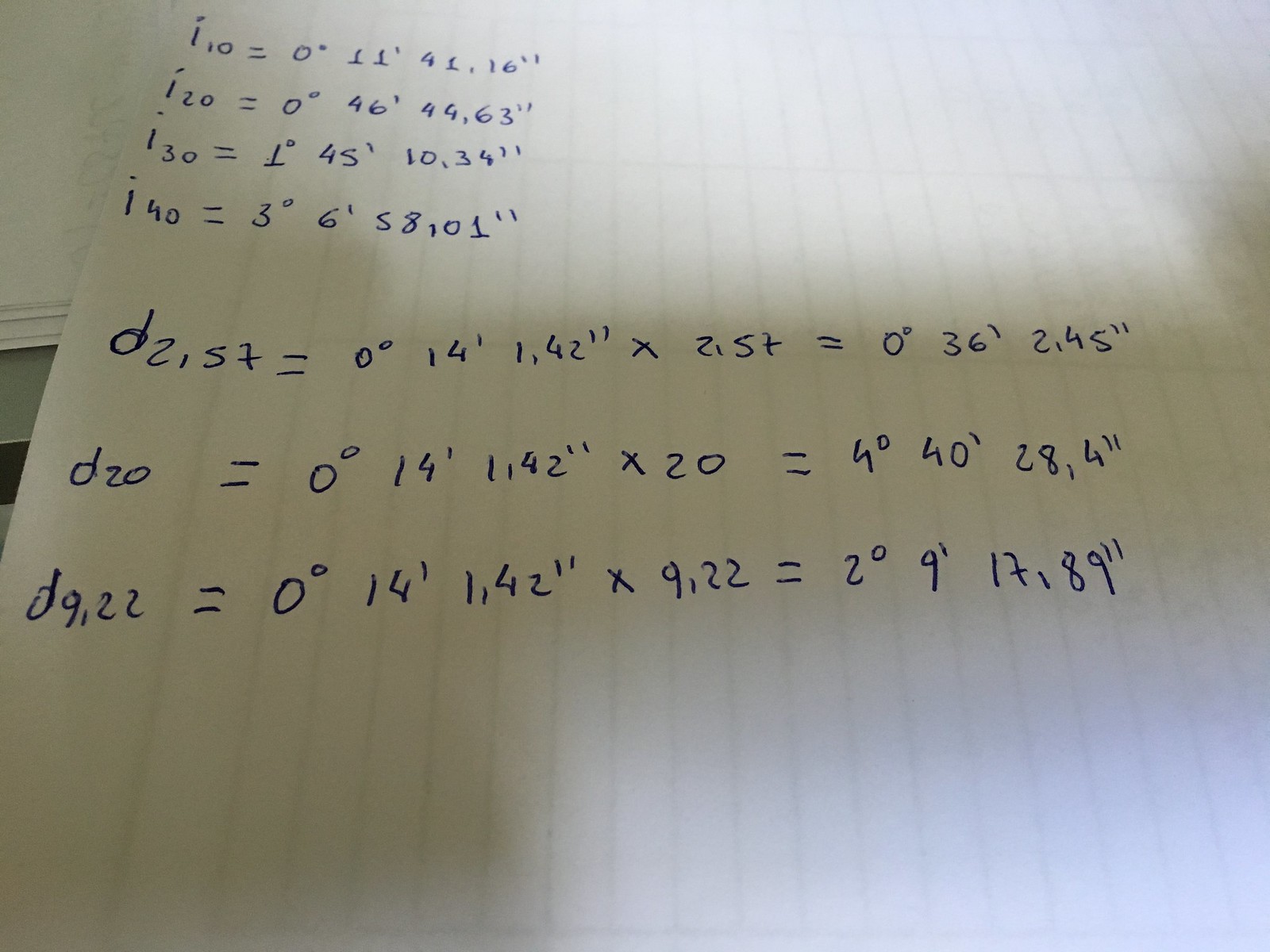A sheet of paper, likely from a notebook or loose-leaf pad, is positioned in the image. The paper is lined with faint grayish or possibly very light blue lines. The text on the paper resembles algebraic equations but could span other mathematical disciplines. 

On the top half of the page, there are four lines of equations, beginning with the variable "I-" followed by increments of ten: I-10, I-20, I-30, and I-40. Each line features an equation with various numbers following an equal sign. These equations occupy approximately one-third of the page.

The bottom half of the page presents three more equations centered around the variable "D." These are more complex, featuring dual equations with additional measurements and variables. For instance, the first one reads: D2, ST = 0 degrees, 14 feet, 1, 42 inches; times 2, ST = 0 degrees, 36 to the first power, 2, 45 inches. The format is consistent in the two remaining equations, with each beginning with the variable "D" and containing multiple equal signs and numbers.

The overall structure suggests a detailed mathematical or scientific calculation, with both top and bottom sections following a clear pattern involving variables and numerical values.